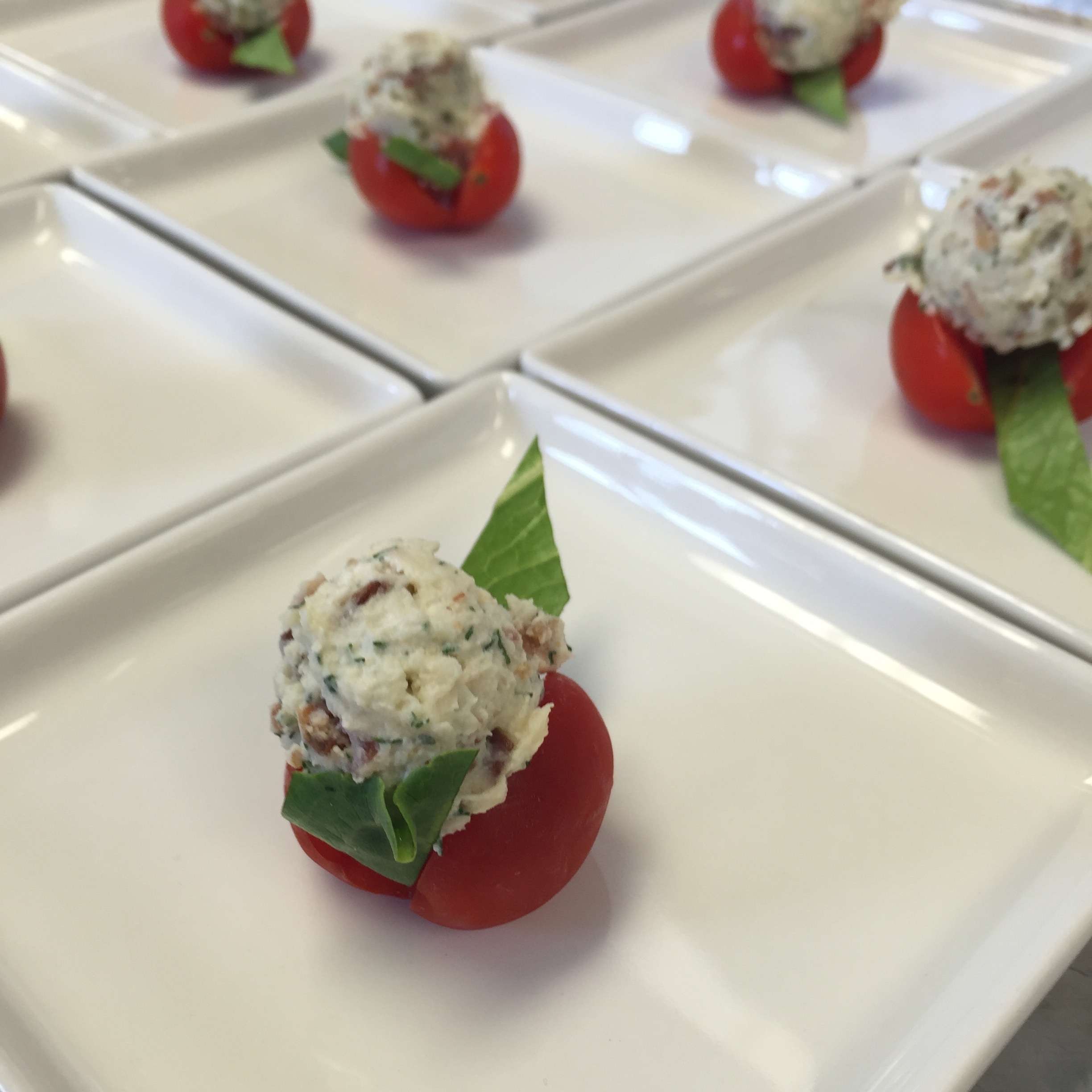This image features a hyper-realistic, angled close-up of several white square plates, each showcasing a meticulously arranged hors d'oeuvre. At the center of each plate, a halved cherry tomato cradles a dollop of creamy white cheese, flecked with herbs. Beneath each tomato, a small piece of lettuce or green vegetable adds a fresh contrast. The creamy cheese has visible green and brown bits, enhancing its gourmet appearance. The lighting from above highlights the vibrant colors and textures of the dish, making the tomato's glossy skin and the cheese's smooth texture stand out. Plate after plate is carefully staged, ready for an event, though those in the background are slightly out of focus, emphasizing the detailed presentation of the front and center plate.